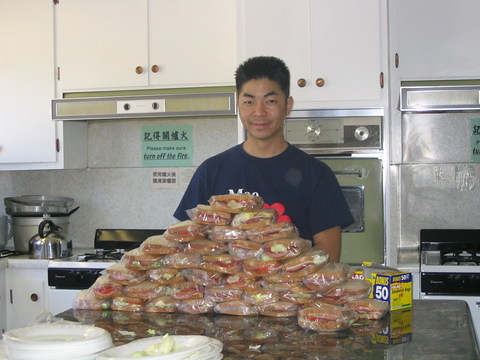In the photo, an Asian man with short, spiky black hair and a medium-light complexion stands in an old-fashioned kitchen, sporting a navy blue t-shirt with a partially visible red logo and white writing. Smiling, he is positioned behind a kitchen island with a glossy brown and green marble countertop, which is dominated by a large, pyramid-like stack of sandwiches. The sandwiches, wrapped in clear plastic bags, number around 30 to 40 and have visible fillings of red and tan, possibly tomato and cheese or salad. Next to them are white styrofoam plates. To the right of the sandwiches, there's a blue and yellow box of GLAD bags, indicating a bonus of 50 bags. The background reveals white kitchen cabinets with dark knobs, an old-style gas stove with burners and a vent hood, a tea kettle, and large silver pots. Above the stove, there are different signs written in Chinese or Kanji, along with an English sign instructing to "please make sure turn off the fire." Additionally, an avocado-green wall oven and other appliances are visible, suggesting a mix of dated, mid-20th-century kitchen decor. The setting, rich with details and kitchen paraphernalia, frames the man who appears pleased, either having made or prepared to serve the sandwiches.